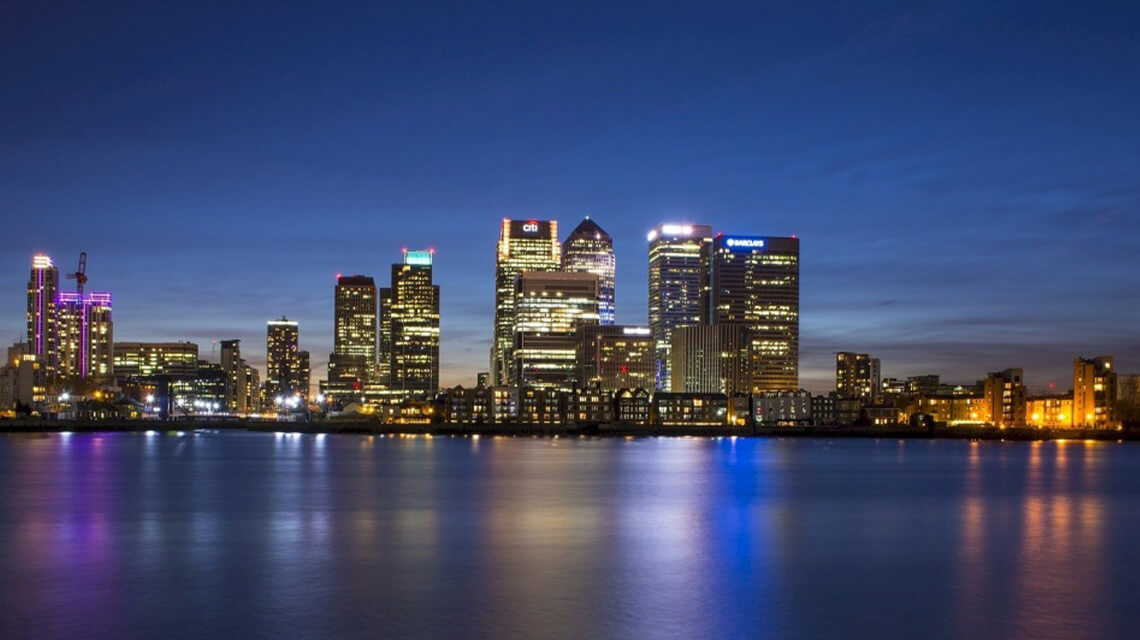The image captures a stunning nighttime skyline of a medium-sized city, with its vibrant lights illuminating the scene. The cityscape, viewed from across a body of water, features a variety of high-rise buildings, although none are exceptionally tall. Among these structures, a prominent "Citi" building stands out. The city’s colorful lights, ranging from yellow to blue, pink, and orange, reflect beautifully off the calm surface of the water, which shows only slight ripples. The sky above is a deepening evening blue, dotted with sparse clouds, and has a faint yellow hue near the horizon, indicating the late hour. In the background, on the right side of the frame, the skyline includes a building with a visible "Barclays" sign. The overall scene is serene and colorful, capturing the city's tranquil yet lively nighttime atmosphere.